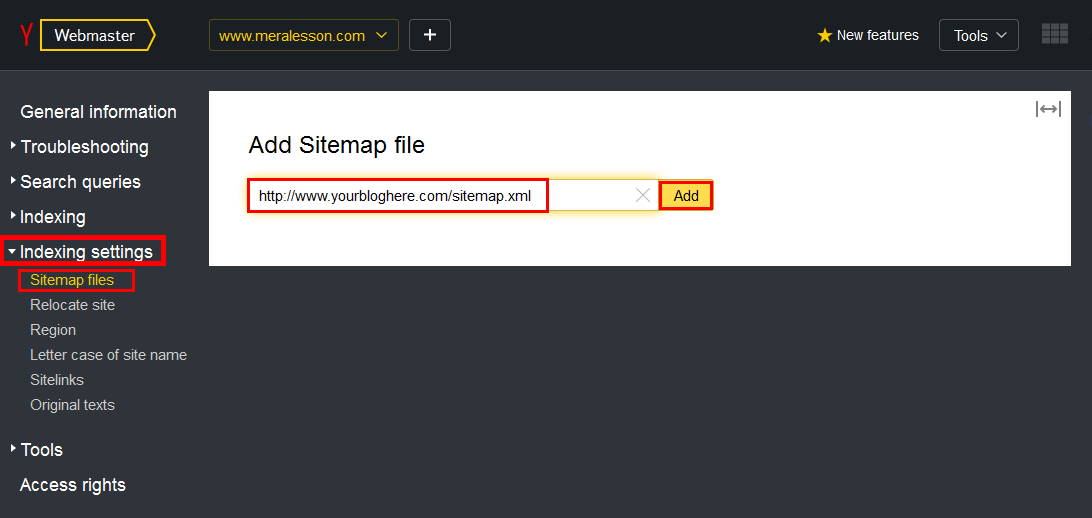This image is a detailed screenshot of a specific webpage interface with a dark gray background and a black menu bar at the top. On the left side of the menu bar, the word "Webmaster" is prominently displayed in white font, enclosed within a gold rectangle that features a pointed end on the right side. Adjacent to this, on the left, the letter "Y" appears in a very thin red font. Following "Webmaster" to the right, we see the website address "www.messon.com" in gold font.

On the left side of the webpage, there is a navigational menu with items listed in white font. The menu includes the following items:
1. General Information
2. Troubleshooting
3. Search Queries
4. Indexing
5. Indexing Select Settings, which is outlined in a red rectangle
6. Sitemaps Files, written in yellow font and also highlighted by a red rectangle

Center-aligned and positioned towards the top, there is a large off-white rectangular section. Within this section, in large gray font, is the instruction "Add Sitemap File." Below this, there is another rectangle containing the placeholder example "http://www.yourbloghere.com/sitemap.xml," indicating where users should enter their actual sitemap file URL to replace the provided example text.